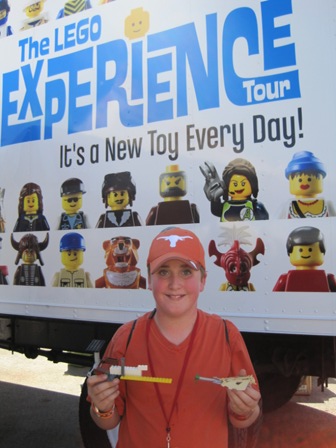This vibrant outdoor photograph captures a young boy, approximately 12 years old, standing near the side of a large, white semi-truck. The boy has a happy smile on his face and is looking up towards the viewer with bright blue eyes. He is dressed in a red v-neck shirt and a matching red hat adorned with a bull symbol at the front. In both of his hands, he holds assembled Lego figures, proudly displaying them. Behind him, the side of the truck features a colorful display of various Lego characters along with a prominent blue-lettered banner that reads, "The Lego Experience Tour." Beneath this banner, in black text, is the tagline, "It's a new toy every day." The photograph is meticulously composed in portrait orientation, with a focus on the detailed realism of the scene.